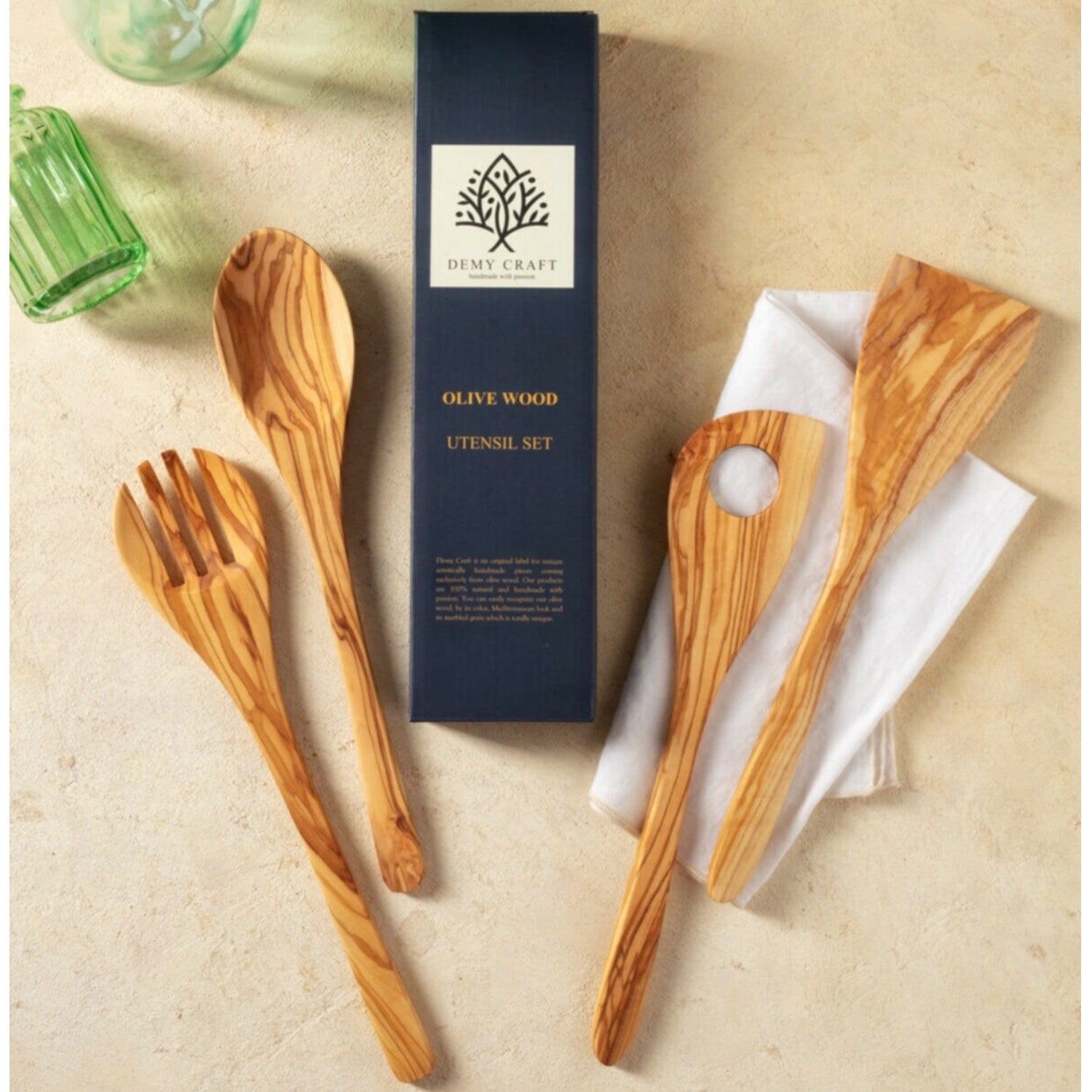In this detailed promotional photograph for the Olive Wood Utensil Set by DemiCraft, four distinct wooden kitchen utensils are showcased. The set includes a fork and spoon, likely intended as a salad serving set, both made from polished, shiny olive wood with a bamboo-like pattern. These are positioned on a light sand-colored table surface. On the right side, a slotted stirrer and a spatula, also crafted from olive wood, rest on a pristine white cloth napkin. At the center of the arrangement is the product packaging, a deep blue box adorned with gold writing and an ivory-colored logo featuring a tree. The image is accentuated by two jade green glass items located in the upper left corner—one a jar, the other resembling a glass orb. All elements are set against a beige, marble-like countertop, creating an elegant and inviting presentation perfect for a promotional shot intended to highlight the utility and aesthetic appeal of the utensil set, making it an ideal gift option.